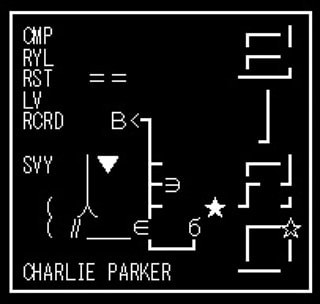The image depicts a black rectangular box with a white border. In the center, there are various white shapes and symbols, resembling a digital diagram or a circuit. Notable features include a sequence of letters in the top left corner: "CMP R-Y-L R-S-T L-V R-C-R-D" followed by "S-V-Y." The bottom left corner prominently displays the name "Charlie Parker." There are several lines and arrows, some forming sideways 'L' shapes, scattered across the right side. In the middle, among various symbols, there is a combination "36EB." Additional elements include stars and a white downward triangle, further contributing to the intricate and possibly technical design of the image.